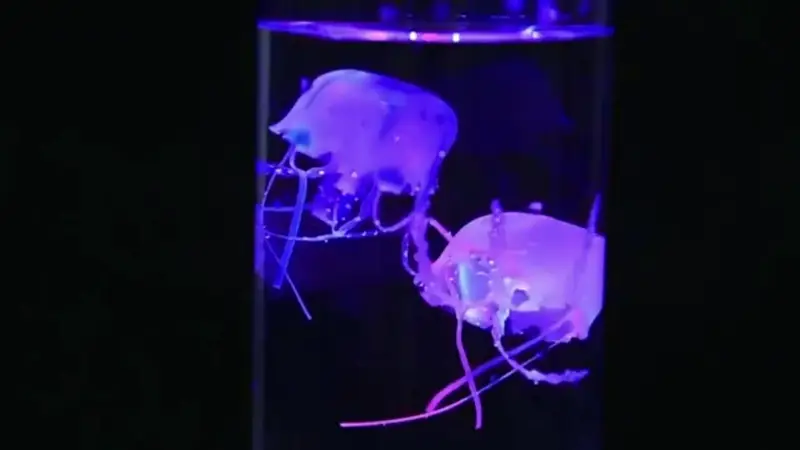This up-close photograph features a cylindrical glass tube, centrally positioned against a completely pitch-black background. Inside the clear container, two jellyfish, illuminated in striking neon hues of blue and pink, gracefully float. Their semi-translucent, half-moon shaped bells crown their delicate, skinny tentacles, which extend downward in elegant patterns. The jellyfish are arranged with one slightly above the other, and each sports four to five slender tentacles. The tube appears to be filled with clear water, and the top of the container is faintly visible, enhancing the scientific specimen appearance of the scene. The illumination from the jellyfish creates a mesmerizing contrast against the dark backdrop, casting a fluorescent purple and blue glow that highlights the ethereal beauty of these vibrant sea creatures.